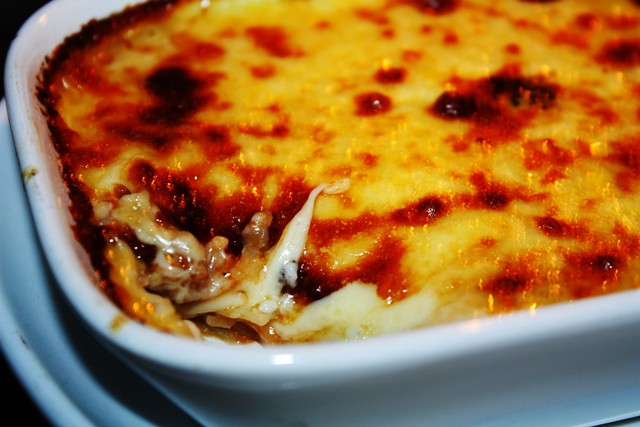A close-up shot captures a delectable-looking Italian dish, likely lasagna or perhaps eggplant parmesan, baked in a white ceramic Pyrex dish. The dish is generously covered with melted cheese and sauce, with some cheese showing enticing dark brown crusts and slightly burnt edges, adding to its savory allure. A portion has been scooped out from the left-hand corner, revealing the saucy, cheese-stretching layers underneath. The Pyrex dish sits on a bluish-bordered mat, adding contrast to the vibrant colors of the food. The overall presentation, with its shiny, golden-brown cheese resembling a perfectly cooked pizza topping, makes the dish look incredibly inviting and delicious.